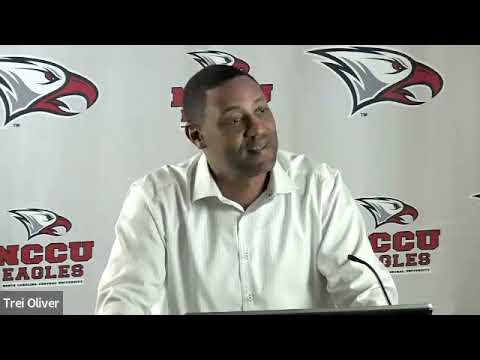In this photograph, a dark-skinned man with very short hair stands behind a podium, speaking into a microphone attached to it. He is wearing a long-sleeved, white button-up shirt and appears to be addressing an audience. The background is filled with a white banner featuring multiple images of an eagle's head, with red beaks and tongues, oriented to the right. Below the eagle illustrations, in bold red letters, it reads "NCCU Eagles." The lower left corner of the image has an edited caption in gray with white letters stating the name "Trey Oliver." The photograph is framed by two narrow black horizontal strips at the top and bottom, adding a distinctive border to the composition.